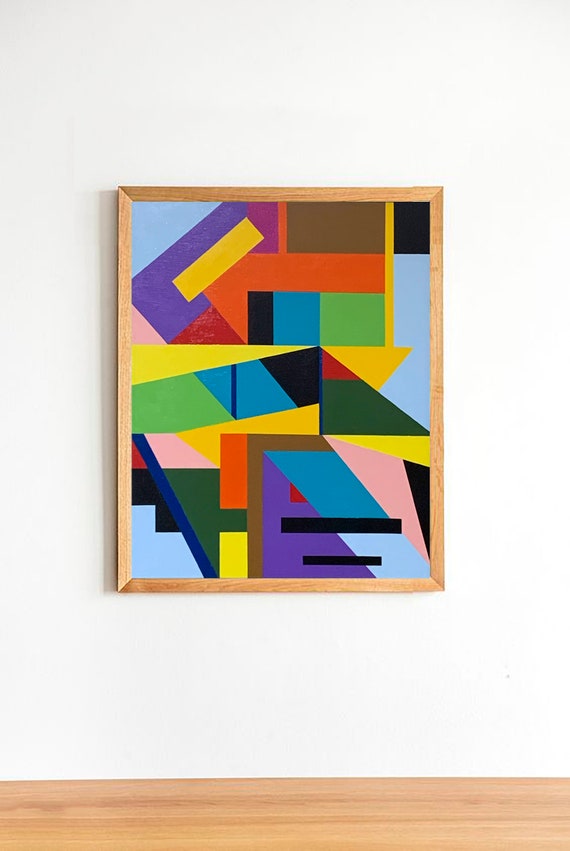The image features a vibrant abstract painting, rendered in a modern, Picasso-esque style, prominently hanging on an off-white gallery wall with a light wood floor below. The painting is framed in a light blonde wood that complements the flooring. The composition is rich in geometric shapes, including triangles, squares, and rectangles, arranged in an evocative, non-representational pattern. A myriad of vivid colors, including purples, yellows, blacks, oranges, reds, blues, greens, fuchsias, and pinks, create a dynamic visual tapestry. Notably, a staircase-like pattern appears at the bottom left, while the right side of the painting hints at a face-like structure with a red triangular eye, a large horizontal black rectangle for a nose, and another black rectangle beneath it representing a mouth. The piece exudes a sense of movement and complexity, inviting viewers to explore its multifaceted design and color interplay.